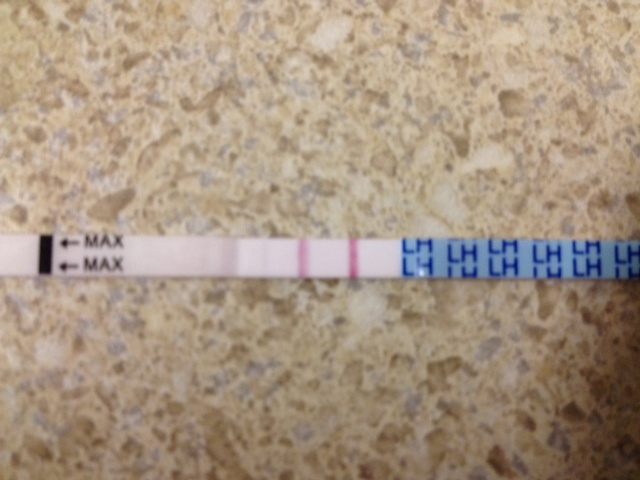The image depicts a COVID-19 test strip laid out on a beige and white marble-like countertop, possibly located in a kitchen or bathroom. The entire length of the test strip spans the photograph. On the right-hand side of the strip, there is a blue section which features the letters "LH" continuously repeating. On the opposite end of the strip, near the edge, a bold black line is visible, followed by the word "MAX" written twice consecutively with small arrows pointing towards the black line. Moving towards the blue end of the strip, the test result area is encountered, characterized by a white backdrop adorned with two red lines. The red line on the left is noticeably fainter than the more vivid red line on the right, yet both lines are distinctly visible. This result signifies a positive test for COVID-19.